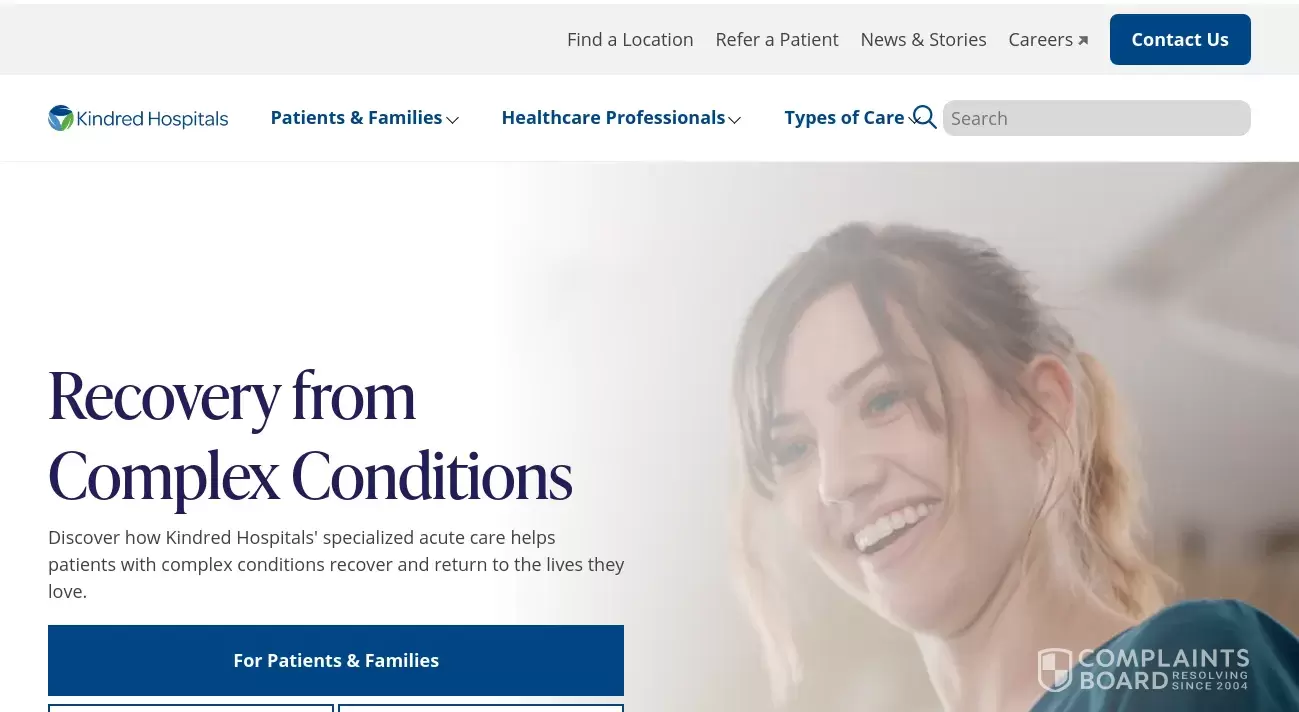The screenshot captures a section of a hospital website, presumably for Kindred Hospitals. The header features a thin purple strip with navigation options like "About Us," "Careers," and a small house icon for the homepage. Below this, a white strip displays the green and blue Kindred Hospitals logo, accompanied by the text "Empowered by Sky on Health." The text also indicates that users can talk to a registered nurse by calling 1-866-KINDRED or 1-866-546-3733, with the number in blue and black.

Further down, a navy search box featuring a magnifying glass icon is available for users to search the site. A blue strip beneath it has white text listing "Our services," "Find a location," "For healthcare professionals," and "Contact us."

The main section shows an image of an African-American woman, middle-aged or older, with curly black hair and a tracheotomy tube, indicative of medical treatment. Parts of two medical professionals are visible: the elbow of a doctor in a white lab coat and the back view of another woman.

Adjacent to the image is a blue and white box stating, "We're committed to healing, recovery, and an exceptional patient experience." Another box nearby explains, "Kindred Hospitals' expert caregivers work to exceed the expectations of you and your loved ones on your recovery journey."

A purple box below features text in white, black, and orange that reads, "Find a location near you." Two white boxes invite users to search by location name, city, state, or zip code, and to filter by specialty hospitals, the latter featuring an orange pull-down arrow. An orange and white button labeled "Search" is prominently displayed for initiating the search.

Overall, the image presents a detailed snapshot of a user-friendly hospital website focused on patient care, accessibility, and support.